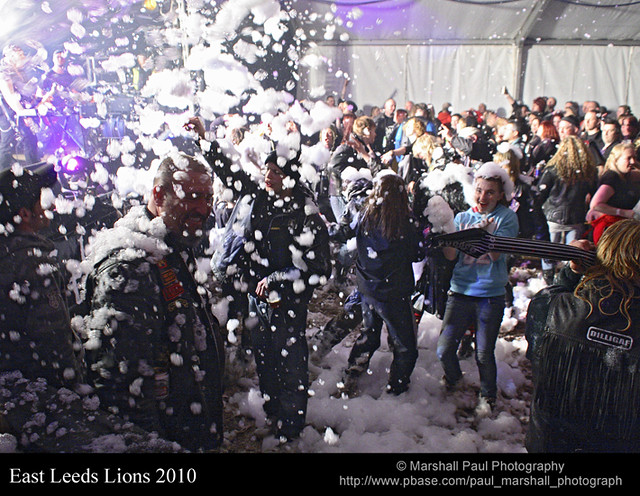The image depicts a lively indoor scene with a large group of people gathered in the center, all smiling and laughing as they get covered in bubbles and foam. The event appears to be taking place inside a large, tent-like structure with white and gray walls, and there is a vibrant purple light shining from the left side. The crowd is illuminated by an array of colors including black, white, gray, light blue, red, purple, yellow, and orange. At the bottom of the photograph, a black banner runs across the screen, displaying white text that reads "East Leeds Lion 2010." It is noted as the work of "Marshall Paul Photography," with corresponding website information: http://www.pbase.com and http://www.paul-marshall-photographs.